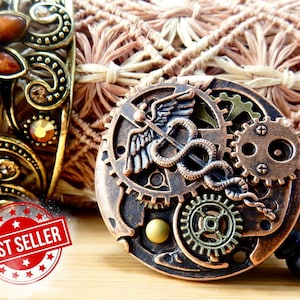The image depicts a steampunk-themed product displayed on a light brown wooden table. In the lower left corner, there is a red circular emblem with white text proclaiming "Bestseller," adorned with small stars around its edges. The focal point is a circular metallic object on the right, detailed with bronze and copper gears, evoking the intricate inner workings of a watch or clock. It features the medical caduceus symbol prominently on its surface. To the left of this metallic object is what appears to be a decorative gold bracelet with brown beads and small jewels, possibly draped over a yarn-like or thread-based material. In the background, there is a larger object, perhaps a bag or bottle, embellished with spiral floral designs and pink and white thread-like structures, complemented by metallic elements of gold and silver along with brown stones and intricate gold work. Overall, the photograph showcases a collection of finely crafted and intricately detailed items, though the exact nature of the central metallic piece remains ambiguous, evoking interpretations ranging from a belt buckle to a decorative artifact.